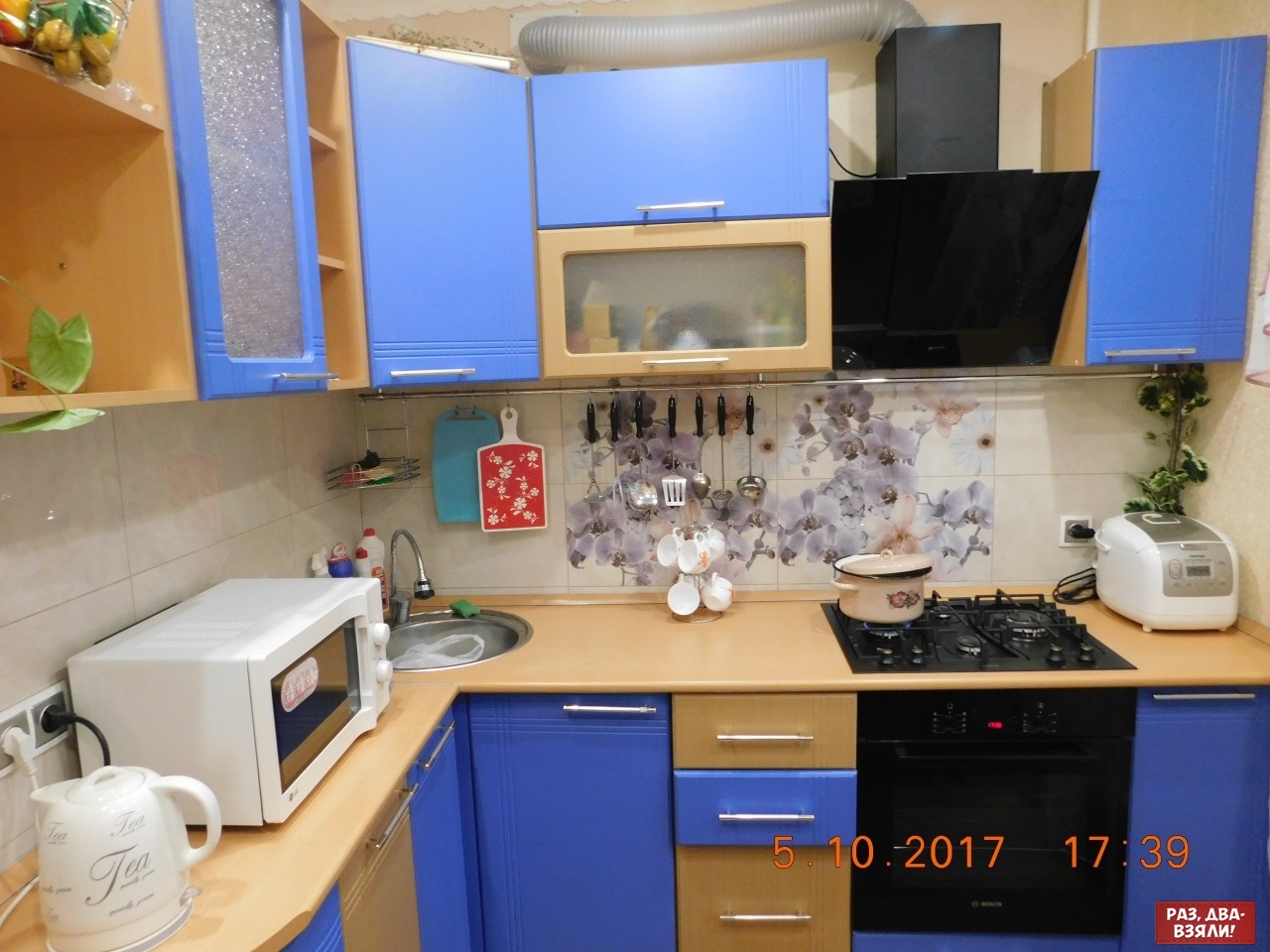This is a detailed photograph of a kitchen taken on the 5th of October, 2017, at 17:39, as indicated by the date and time stamp on the image. There are Russian characters encased in a small red box located at the bottom right corner of the image. The kitchen is furnished with blue cabinets that feature silver handles, interspersed with sections of light brown wood. The countertop is brown, extending in an L shape where the two countertops meet, which houses a small circular sink.

To the right of the sink, a black stovetop with a cream-colored pot sits beside a black oven and range hood. Near the stovetop is a rice cooker, and adjacent to it is a green plant providing a touch of nature. On the left-hand side, there's an electric tea kettle with "tea" written on it, a toaster oven, and a white microwave. The backsplash is decorated with images of purple flowers, contributing to the aesthetic charm of the kitchen. Additionally, cutting boards and various cooking utensils are seen hanging on the wall, enhancing both the functionality and the visual appeal of the space. The cohesive placement of appliances and decorative elements creates a warm, inviting atmosphere in the kitchen.